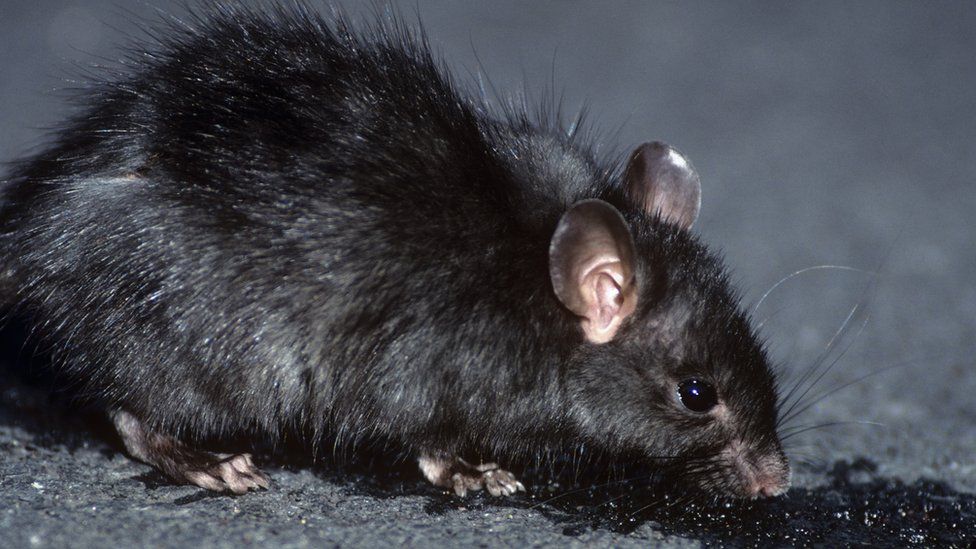This image is a close-up photograph of a very cute black mouse or rat, captured in profile, facing to the right. The animal's fluffy black fur covers most of its body, with the exception of its small, rounded ears which are black on the tips but possess a pink, lighter skin inside. Its black whiskers sprout from a small pink nose that seems to be either sniffing or licking something on the gray ground below. The photograph reveals the right side of the animal, showing its black eye and distinctive fluffy fur. You can also see its pink-tipped feet, lightly touching the flat, gray cinder block or stone surface. The scene includes a scattered arrangement of blackberries or seeds near the lower right corner, which the mouse is likely investigating or eating. The background appears blurry, composed of shades of gray and black, resembling a street or dark asphalt, enhancing the focus on the adorable rodent and its actions. Light reflects inside its right ear, accentuating the lighter skin color within, adding to the detailed charm of this image of the inquisitive, black-furred creature.